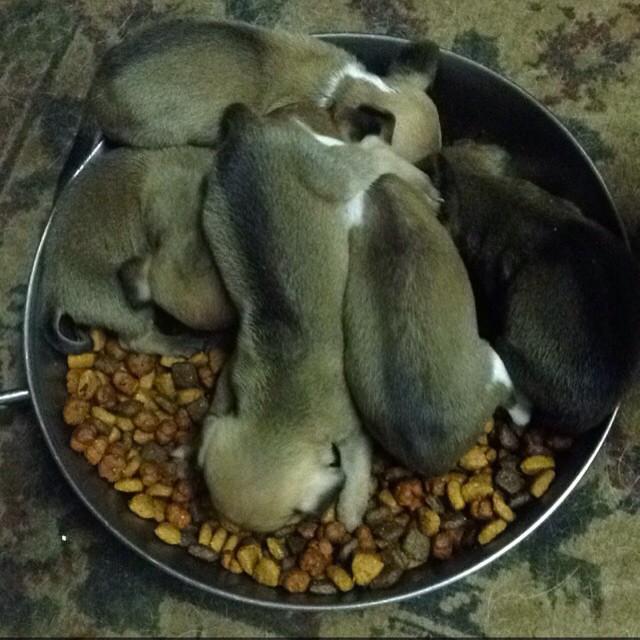The photograph captures a heartwarming scene of five newly born puppies gathered in a large, sterling silver bowl filled with multicolored dog kibble, ranging from mustard yellow to dark brown. The bowl, equipped with a handle, is placed on a beige marble tiled floor with black highlights. The puppies, seemingly only a few weeks old, are a mix of dark brown, grayish, and black with hints of white. A distinctive puppy in the center, sporting a black stripe down its back, stands out as it sprawls over its siblings, all eagerly munching away with their tiny faces buried in the food. Despite their small size, the puppies are fully contained within the bowl, each immersed in a communal meal, radiating an excited and happy energy. The background subtly features a throw rug or carpet adorned with green and burgundy floral designs, adding a cozy touch to the charming tableau.